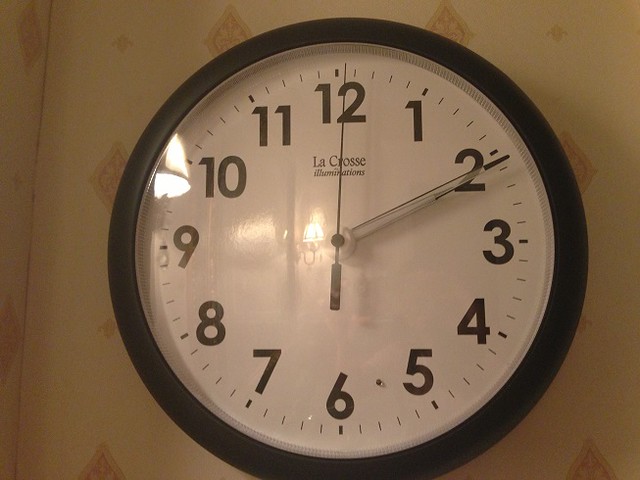The image depicts a close-up of a wall clock with a black border and a white face featuring black numerals from 1 to 12. The clock reads 10 minutes past 2 o'clock, with the hour and minute hands pointing at the 2 and a thin black second hand ticking near the 12. The clock face prominently displays the brand name "La Crosse Illuminations" in the center. A light source from the room is reflected on the clock’s glass cover, and the clock casts a subtle shadow to the right. The clock is mounted on a wall covered in beige or tan wallpaper with diamond-shaped patterns. Additionally, two lamps from elsewhere in the room are faintly visible in the clock's reflection.